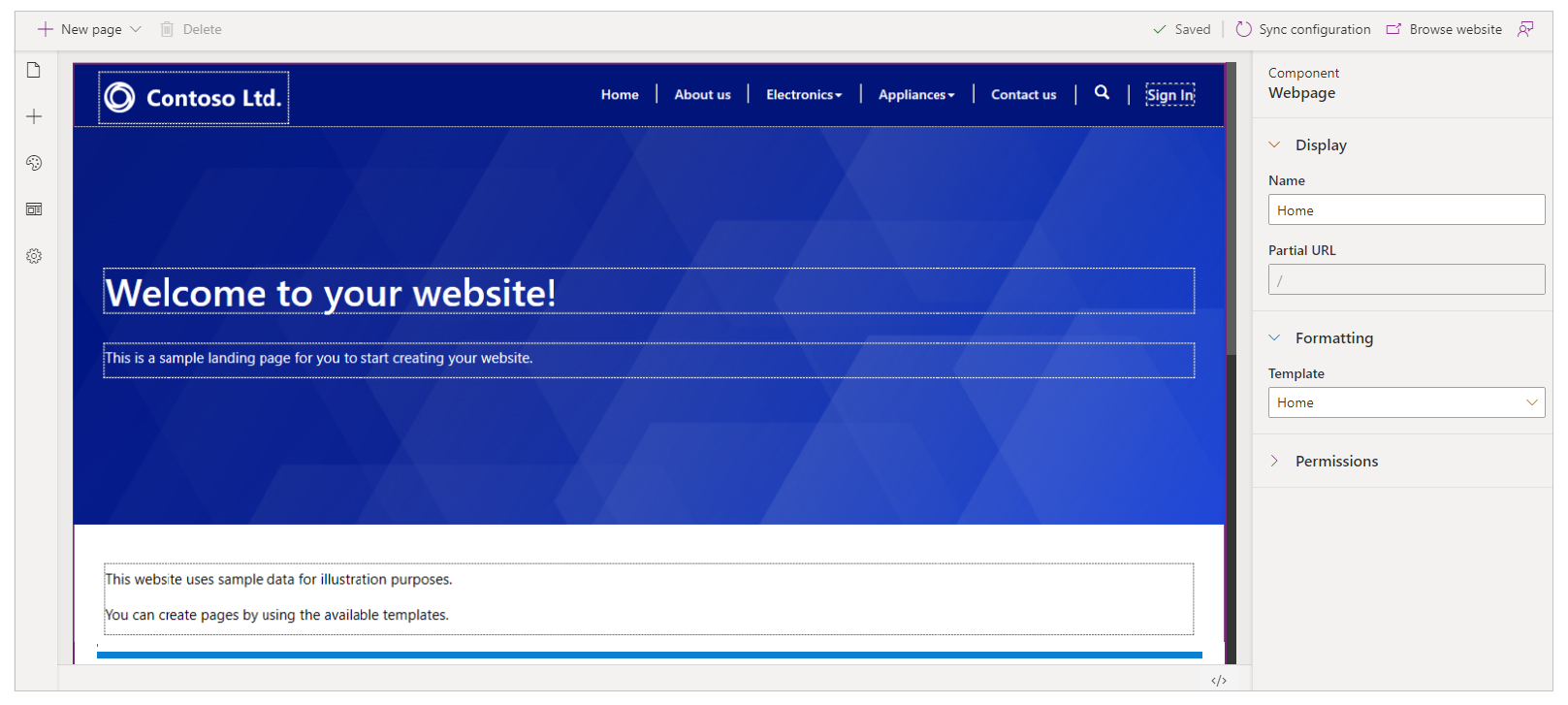This screenshot captures the interface of the ContosoLTD website creation tool. Dominating the top left corner is a "+ New Page" button, depicted as a folded paper icon symbolizing a new page creation. Below this, a vertical toolbar features a sequence of buttons: a plus sign, a gear icon at the bottom, and two indistinct icons in between, one circular and the other square.

On the right side of the interface, the top right displays the label "Component Web Page," indicating the active project. Below this label, "Name: Home" signifies the current page being edited, identified as the home screen. The interface includes fields for a partial URL and template options, showing that the "Home" template is in use.

The design of the main workspace is predominantly blue, featuring a striking blue diamond pattern at the center. White text on this background welcomes users with the phrase, "Welcome to your website." This clean, blue-themed layout offers a basic yet inviting introduction to the newly created web page.